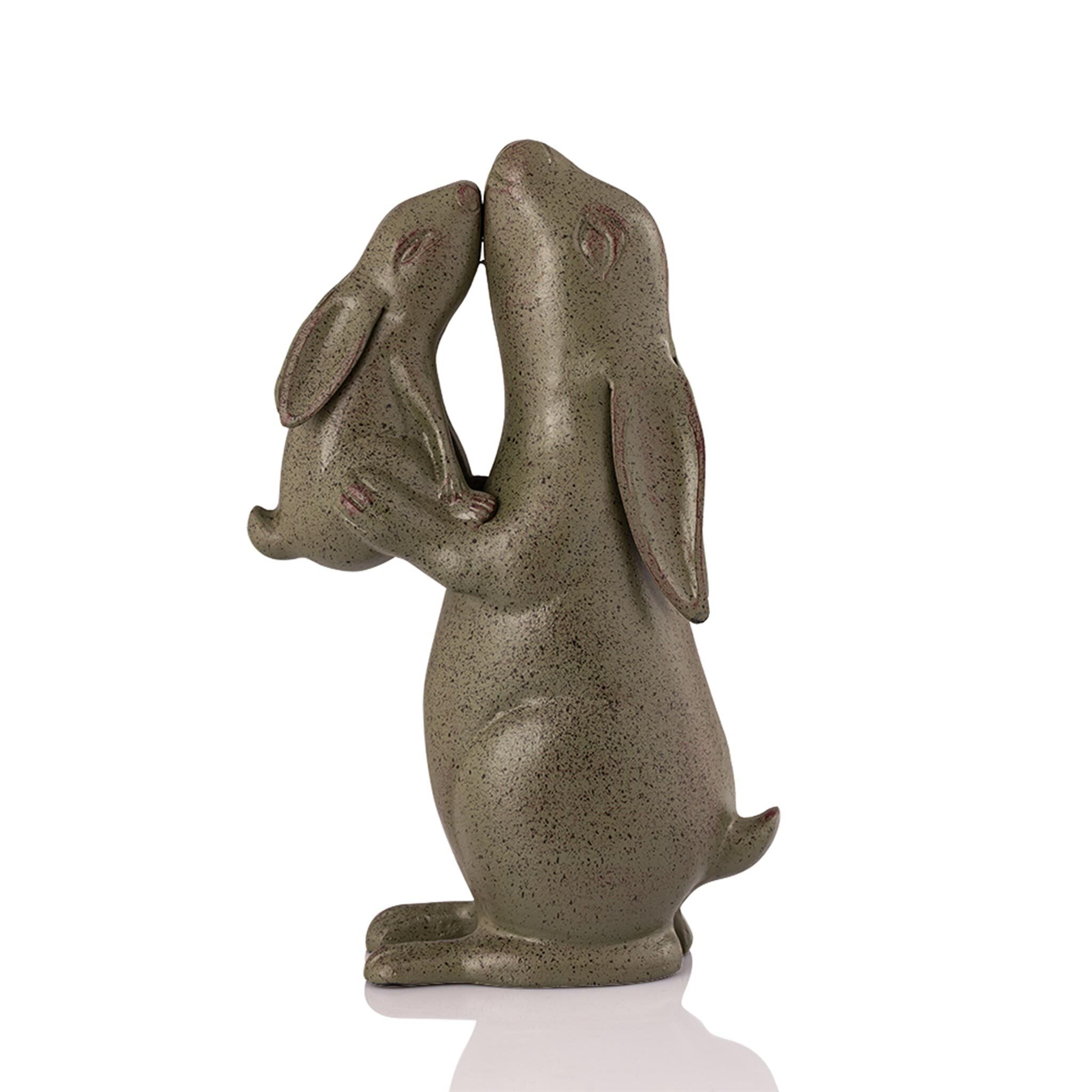The image presents a photographic depiction of a grayish-brown stone sculpture set against a stark white background. The central focus is a large rabbit figurine, standing upright on its hind legs, and looking upward. This larger rabbit, featuring long, tapered ears, and a distinctively curved tail, embraces a smaller rabbit in its front paws. The smaller rabbit, also detailed with elongated ears and a matching curved tail, nestles affectionately against the larger rabbit, with both rabbits' heads joined together as they gaze upward. A shadow cast by the sculpture on the surface below adds depth to the scene. The refined craftsmanship captures the tender moment of the two rabbits, evoking a sense of warmth and familial bond.